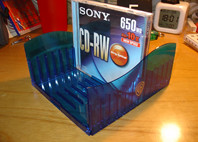The image depicts a laminate wood desk featuring an old Sony CD-RW prominently placed in the middle of a translucent blue wave-like plastic CD holder that can accommodate up to 12 CDs. The CD itself displays "Sony" in white letters, "650" in white, and "10x" in orange. In the background, there is a white digital clock displaying the time "18:01." The desk also holds a couple of books, one of which is distinctly red, along with other miscellaneous cluttered items.